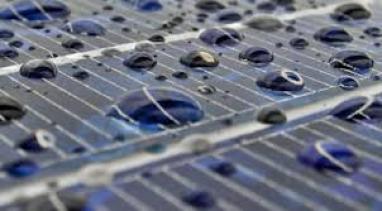This is a highly detailed, color close-up photograph of water droplets on the surface of a solar panel. The panel's surface is a blackish-blue color, interspersed with several large horizontal metallic lines and smaller vertical metallic lines. The array of water droplets, numbering a couple dozen, ranges in size from very large to tiny specks. These droplets magnify the underlying metallic lines and create distortions that reflect the light, amplifying the pattern of the panel. Some droplets appear black or blue, highlighting the intricate interplay of color and texture on this plastic-like surface.